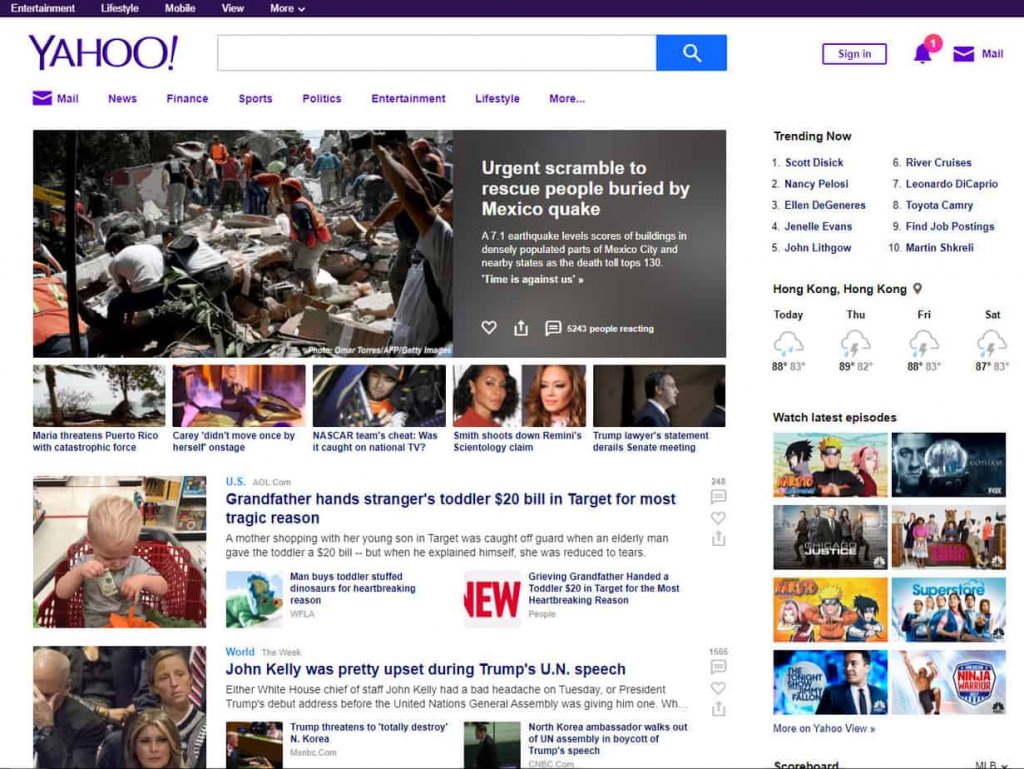This image is a cropped screenshot of the Yahoo! main page as displayed on a desktop. The background of the page is white, lending a clean and modern look to the interface. 

At the top left corner, there is the Yahoo! logo prominently displayed in large purple letters. Centrally located near the top of the page is an expansive search box. Adjacent to the search box on the right, there is a blue square featuring a magnifying glass icon, which signifies the search function.

On the right side of the page, a vertical panel provides various functionalities and information. At the very top right of this panel are three icons: the sign-in button, an alert button, and the Yahoo! Mail icon.

Directly below these icons, there is a small box titled "Trending Now," divided into two columns. The left column lists the top five trending topics, while the right column lists topics six through ten.

Further down, a section notes "Hong Kong, Hong Kong" with a pin drop icon indicating the user’s location. Following this, there is a small weather forecast section displaying predictions for today through Saturday.

Continuing down the right-side panel, a section titled "Watch Latest Episodes" features eight thumbnail previews for different video content, organized into two rows of four thumbnails each. Beneath these thumbnails, small grey letters state "More on Yahoo! View.”

The main body of the page, on the left, resembles a digital newspaper layout filled with articles. At the top, there is a prominent article with a large thumbnail image. Below this feature article are several smaller article thumbnails aligned horizontally. Lower still are larger rectangular sections with articles presented in a vertical arrangement, guiding the reader down the page in a systematic fashion.